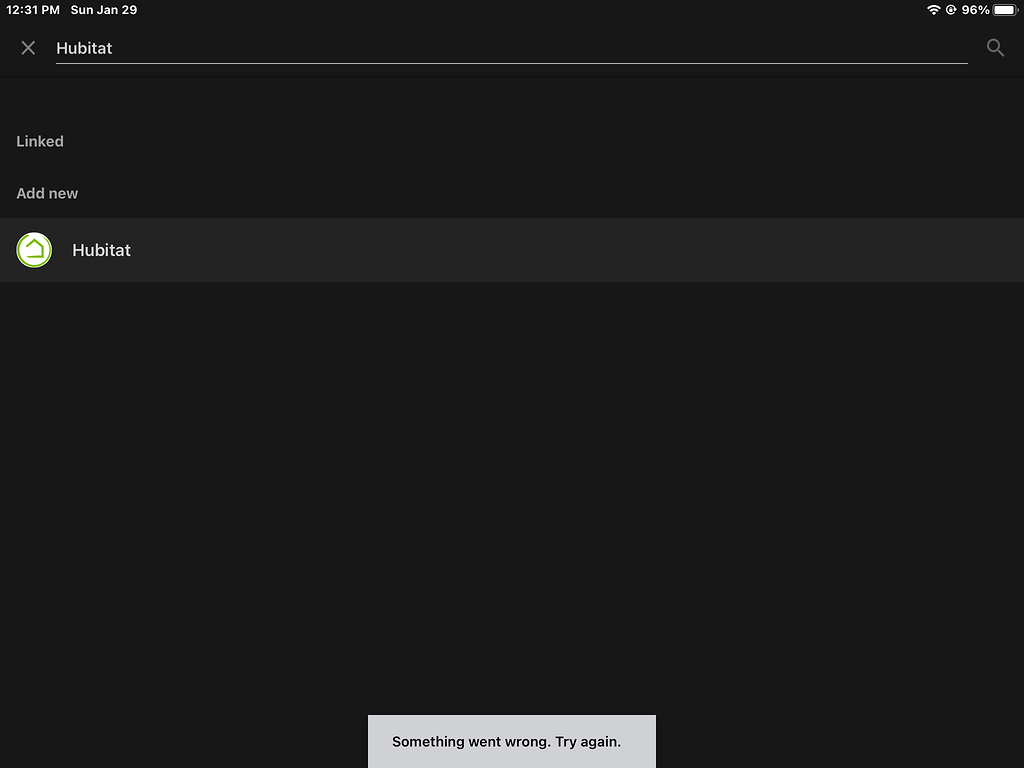The image features a screen capture against a black background with prominent white font. At the top, the status bar displays the time (12:31 p.m.), the day (Sunday, Jan 29), icons for Wi-Fi and battery (showing 96% charged), and the app name "HUBITAT" with a gray 'X' next to it. Below this, there is a thin white line, followed by a gray magnifying glass icon. The text "linked" and "add new" appear in gray. In the center, there is a large black box extending horizontally, with the word "HUBITAT" written inside. A white-and-green circle with a slightly darker green house icon is also present. At the bottom of the image, a gray box contains black text reading "something went wrong try again." The font throughout the image is super bold and easy to read, with excellent image quality and no pixelation or blurring, making it accessible for low vision users.